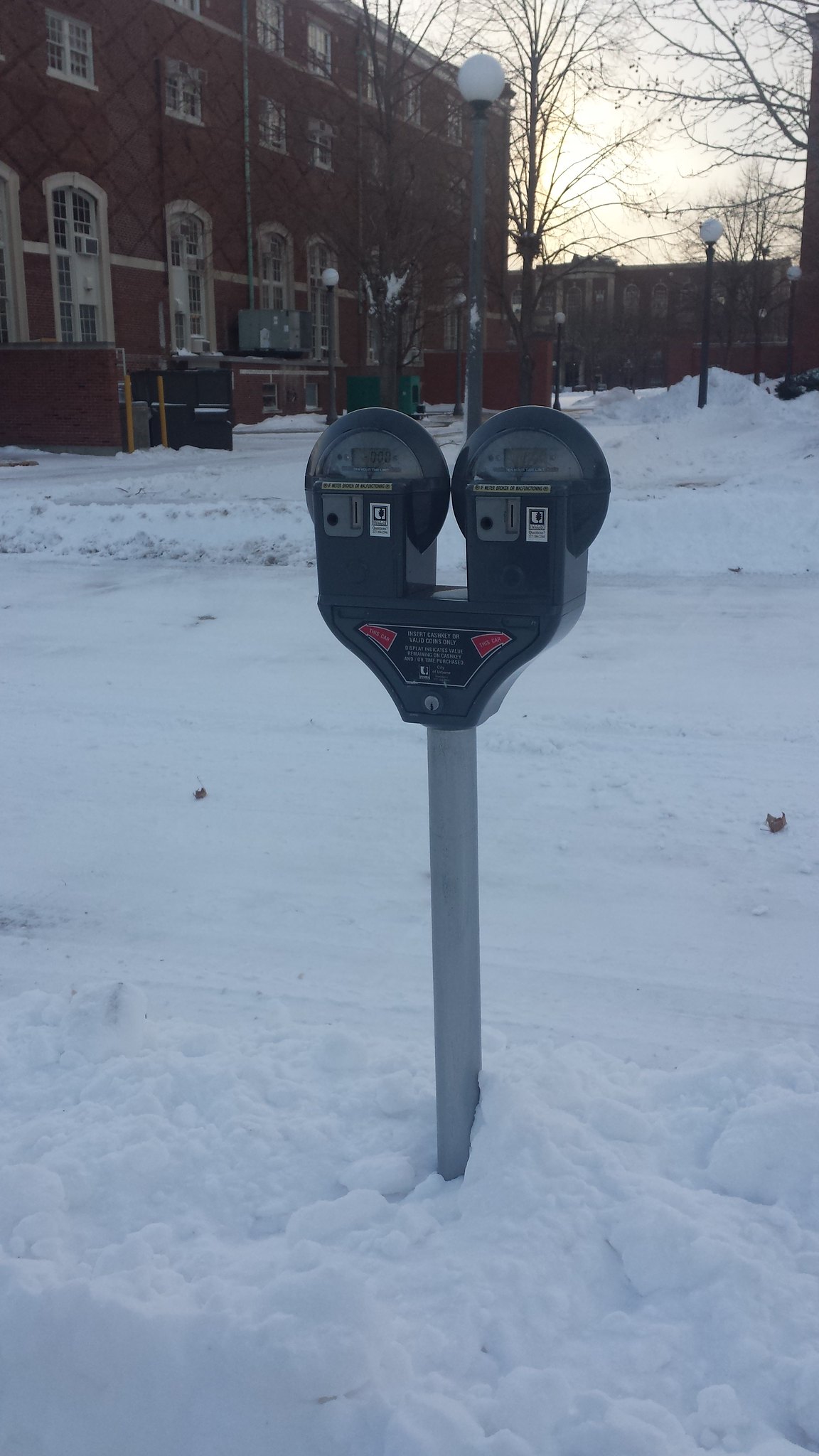In the photograph, we see a snowy winter scene featuring a double-style parking meter, set against a picturesque backdrop of red-brick buildings that appear reminiscent of a college campus. The parking meter, mounted on a pole partially buried in snow, stands prominently in the foreground. It is black and has two sections, each equipped with slots for quarters. 

The surrounding environment is characterized by a thick, snow-covered ground, which appears to have been plowed but still remains heavily packed with snow, creating mounds around the base of the parking meter. 

In the upper left corner of the image, there is a notable dark red brick building with beige-trimmed windows, standing three stories tall. This building is accompanied by another similar structure located in the upper right part of the photo, suggesting a cohesive architectural style likely indicative of an academic setting. 

Additionally, the scene includes some bare trees, their leafless branches silhouetted against a gray, overcast winter sky. There are also round globe light posts and a series of tall windows with white frames, some of which have air conditioners installed. Several sets of stairs lead up to the various buildings, contributing to the urban campus aesthetic. 

Overall, the detailed winter landscape captures a serene yet cold ambiance, with the distinguishing features of the parking meter and the scholarly architecture serving as focal points.